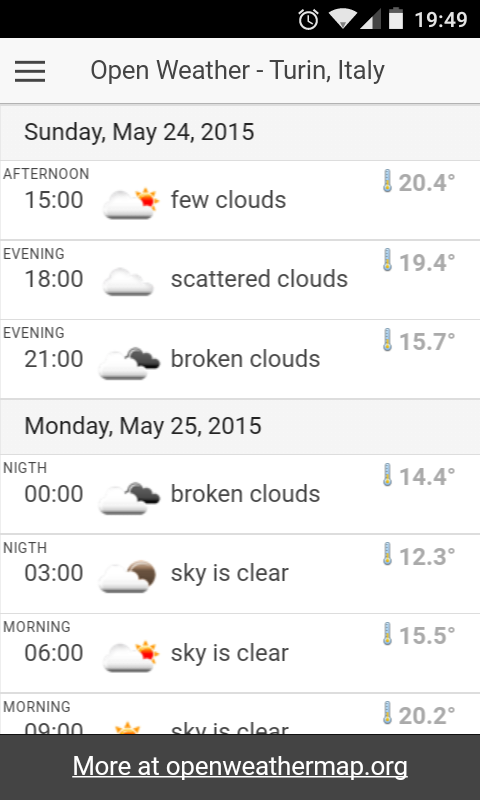This is a detailed screenshot of a weather application on a cell phone, presented in portrait orientation which is significantly taller than it is wide. The image features a white and gray backdrop with a black top border, which includes several status icons: an alarm clock, a fully connected Wi-Fi symbol, a half-filled network connection bar, and a vertical battery indicator showing approximately 80-90% charge. The time displayed is 19:49.

Directly below the black header is a gray box with a thin gray line separating different sections. On the left side of the box is a black hamburger menu icon. The text within this box states "OpenWeather - Turin, Italy." Following this, the date is listed as Sunday, May 24th, with forecast details for the afternoon, evening, and late evening at 15:00, 18:00, and 21:00 respectively. The weather conditions are noted as "few clouds" at 20.4°C, "scattered clouds" at 19.4°C, and "broken clouds" at 15.7°C.

Below this section, the forecast extends to Monday, May 25th, specifically labeled for the "night" period, though misspelled as "NIGTH." The forecast times include 00:00, 03:00, 06:00, and 09:00 hours. The weather for these times is predicted to be "broken clouds" initially, followed by "sky is clear" for the subsequent three periods.